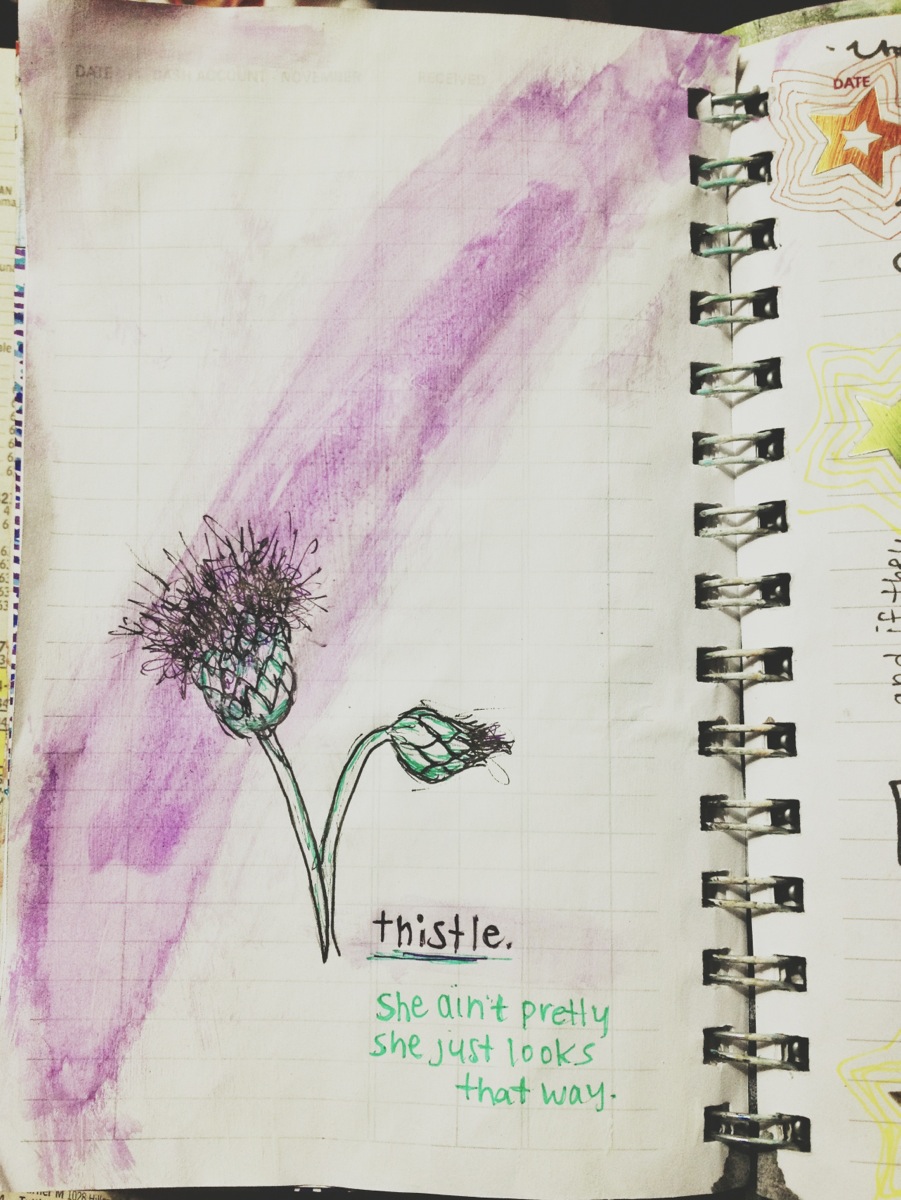A meticulously detailed photograph features a well-used personal notebook, revealing a glimpse into its owner's creative process. The open white page displays a striking purple stripe that spans diagonally from the bottom left corner to the top right. Alongside the vivid stripe, a carefully drawn thistle is prominently labeled with the word "thistle." Below the illustration, an inspirational quote reads, "She ain't pretty, she just looks that way," echoing sentiments of perception versus reality. This notebook serves as a canvas for the owner's thoughts and artistic expressions, encapsulating their unique way of blending imagery and introspection.